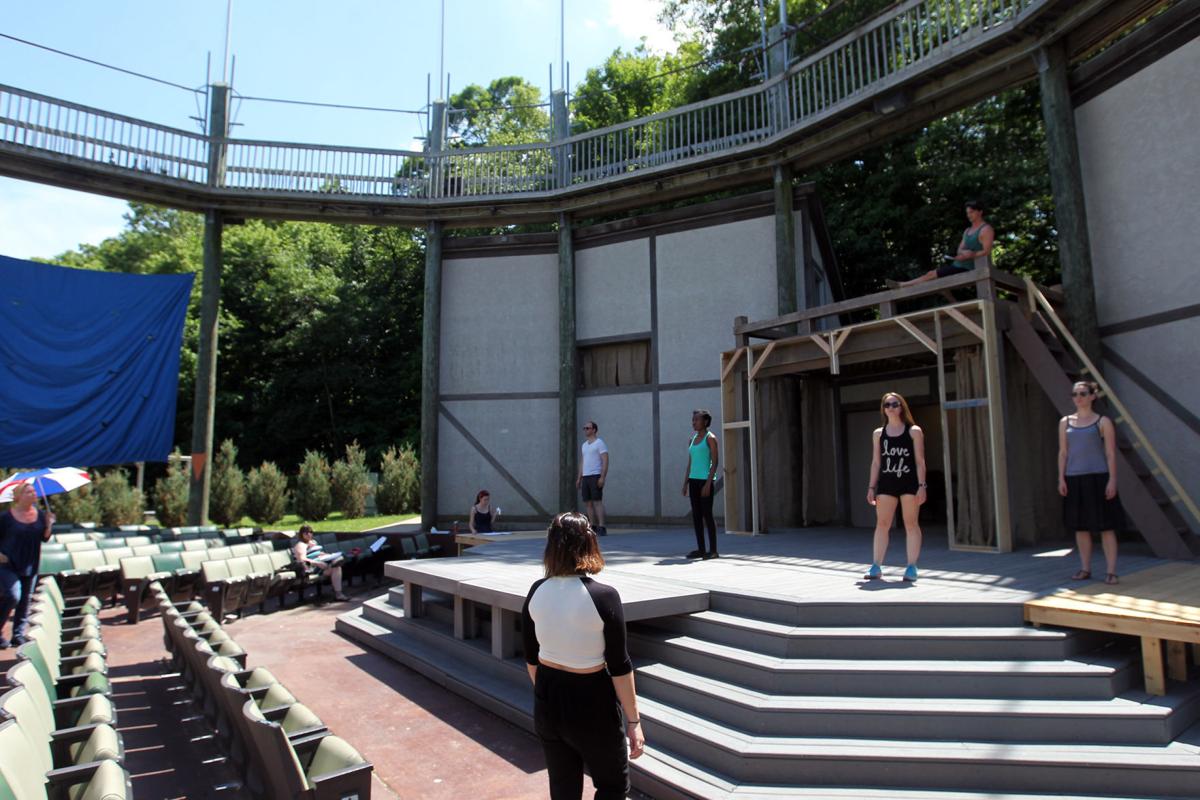This photorealistic image captures an open-air theater set against a lush forest backdrop, featuring a gray, concrete stage with a prominent center platform and ascending steps. Four individuals stand on the stage with their arms at their sides, gazing toward rows of empty green and yellow chairs arranged on the left. The stage is framed by exposed wooden pillars and light gray siding, suggesting a rustic thematic backdrop likely intended for an outdoor Shakespearean play. Above the stage, a man reclines atop a center gate, adding to the scene's dynamic. Suspended beneath an upper walkway border, a blue flag flutters to the left of the image. In the audience, four people are seated, with additional onlookers standing at ground level in front of the stage, enhancing the theatrical atmosphere. The diverse cast includes three females and two males, reflecting a range of ethnicities, actively populating different parts of the staged environment.